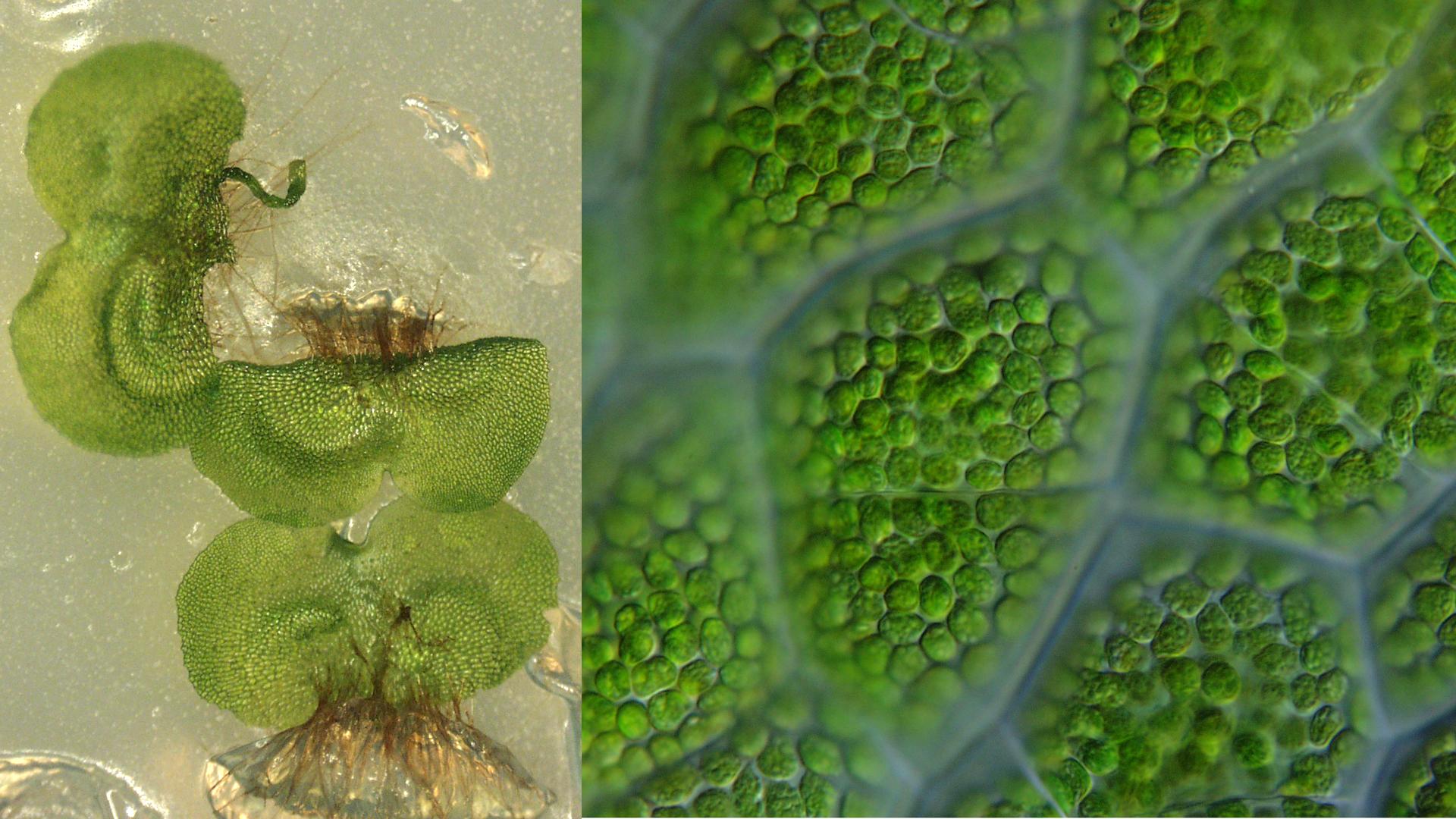The image is a composite photograph featuring two sections, likely taken under a microscope, highlighting intricate cell structures. The left side of the photograph shows what appears to be an oblong, peanut-shaped structure that is light green in color, suggestive of a plant or algae. This structure is embedded in a gel-like or liquid substrate, with numerous small, brown filaments or roots extending from it. Dotted with numerous small green specks, the structure seems to float in a clear liquid medium.

On the right side, the image zooms in on a portion of the left side, revealing a highly magnified view of the cell structure. This section displays a honeycomb-like pattern with distinctly defined compartments outlined in a darker gray hue. Within each of these compartments, numerous bright green dots or ovals completely fill the space, offering a detailed look at the internal composition of the cells. The magnification emphasizes the intricate organization and clustering of these green elements, presenting a vivid exploration of the microscopic world.